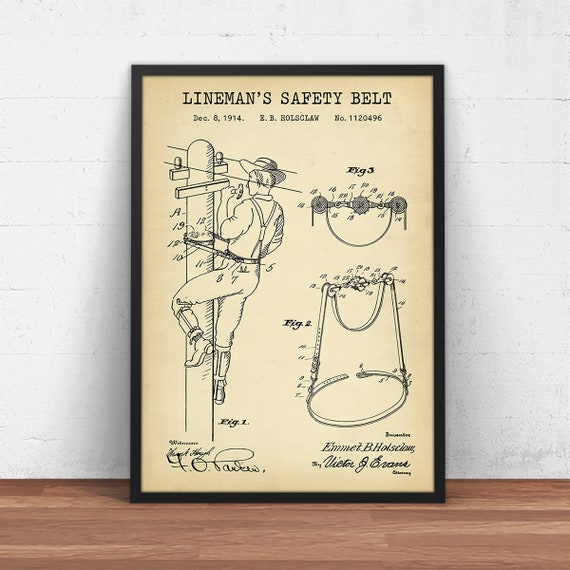This image captures a framed, vintage poster displayed on a brown, wooden surface with a stark white wall as the backdrop. The poster, aged and yellowed, is encased in a sleek black frame and titled "LINEMAN'S SAFETY BELT" at the top in bold, uppercase black letters. Below this, smaller text reads: "DECEMBER 8, 1914 E.B. HOLZKLA NO. 1120496". The left side of the poster features an illustration of a lineman perched high atop a pole, secured by a safety belt wrapped around his waist and the pole. To the right are broken down diagrams, labeled "Figure 3" and "Figure 2", detailing various views of the belt. The intricate details and historical tone of the image are complemented by the signatures in cursive in the lower left and right-hand corners.